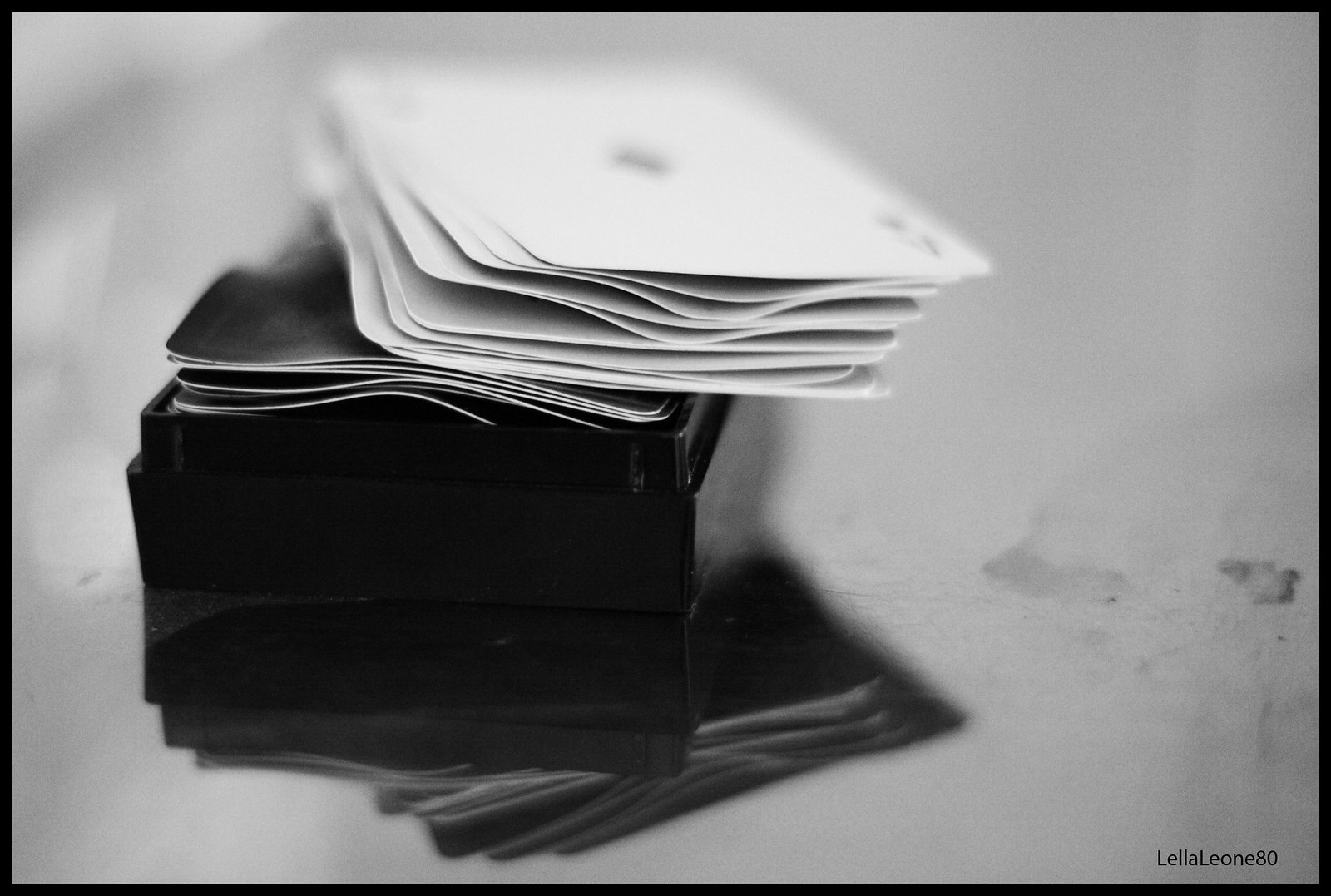Aged and evocative, this black and white photograph is marked in the bottom right corner with the inscription "Lella Leone 80." The photograph itself shows signs of wear, with visible stains and scuffs adding to its nostalgic aura. At its center, warped and weathered playing cards are prominently displayed. The ace of spades lies conspicuously on top of a deck, the cards appearing as if they have been wet and subsequently dried, leaving them distorted and far from flat. These cards rest on an old box, which is brimming with more cards, predominantly facing down and showing a dark back, possibly black. The overall composition of the photograph lends it an artistic quality, intentionally crafted to evoke a sense of decay and timelessness.